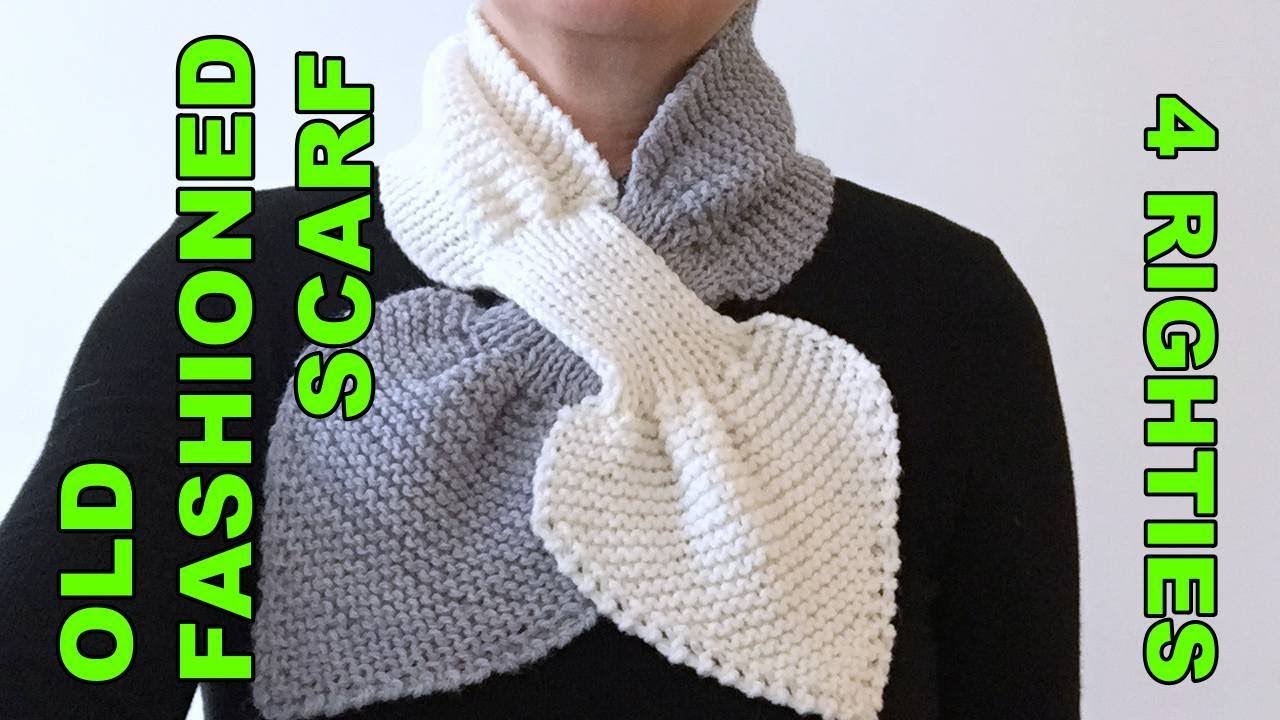The image appears to be an advertisement showcasing a white, possibly crocheted or knitted scarf with a unique design. The central focus of the image is the scarf worn by a person dressed in a long-sleeved black shirt. The individual's face is not shown, with the frame capturing from the middle of their chin to their mid-chest. The scarf, which overlaps at the front, is distinguished by its heart-shaped ends, with one side in white and the other in a grayish hue. The rest of the scarf encircles the neck in white. The background of the image is a plain white. Vertically oriented green text flanks the scarf image—on the left side, the words "Old-Fashioned Scarf" are displayed one word per line, and on the right side, the number "4" is followed by the word "Righties." The text on the left reads from bottom to top, while the right side text reads from top to bottom.